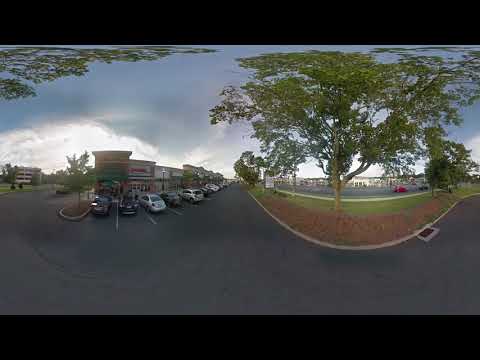This photograph captures an expansive outside area dominated by a parking lot filled with cars, fronting what appears to be a strip mall or a series of stores, with buildings stretching into the distance. The left side of the image prominently displays this blacktop expanse, where a variety of vehicles—including two dark-colored cars, a light-colored car, another dark car, and a silver one—are parked side by side, continuing into the distance until they appear too small to distinguish. Above this scene looms a moody sky, with clouds thickening towards the bottom suggesting a possible incoming storm, transitioning from lighter shades at the horizon to a darker, more foreboding blue near the top.

On the right side of the photograph, a grassy area is bordered by a white line, possibly marking the edge of the parking lot, which features a prominent, green-leafed tree surrounded by smaller trees, suggesting a blend of nature within this urban setting. Additionally, there's a drainage grill visible along the roadway on this side. Further into the background, more roads and buildings are discernible, adding depth to the scene. Notably, a white strip seems to separate the parking lot from a sidewalk or walking path meant for pedestrians. Off towards the left side in the distance, there's a building that could be a multi-story parking garage due to its non-descript exterior.

Overall, the panoramic image blends commercial, natural, and urban elements, all under a varied sky that enhances the composition with its dramatic cloud cover.